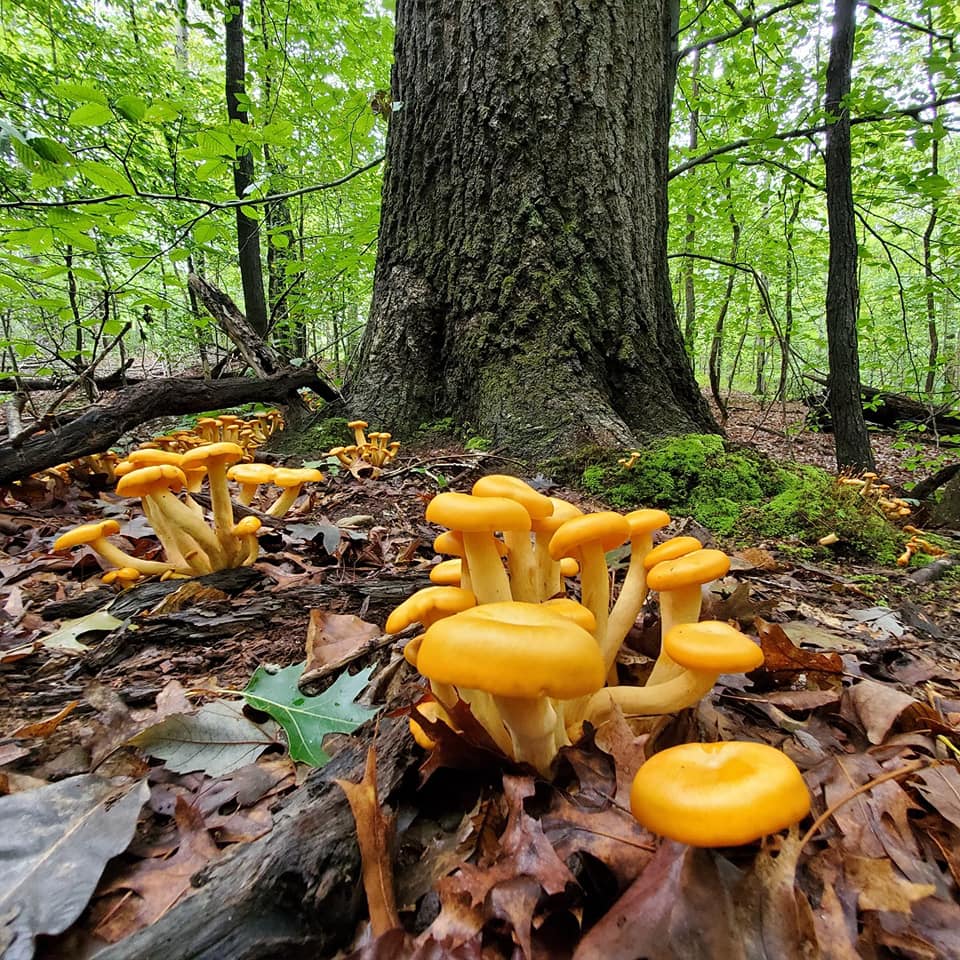The photograph captures an outdoor scene, focusing on a close-up of the base of an old, large tree—likely an oak, given the surrounding leaves. The tree trunk is massive, covered with patches of green moss, and spreads its roots out around it. The ground beneath is strewn with a multitude of leaves, predominantly brown oak leaves, along with some green and yellow ones. Among the leaves, clusters of bright yellow mushrooms with shiny caps and slightly crooked stems stand out. These mushrooms are spread around the tree's base, with some prominently in the foreground and others grouped on the left side and in the background. A dried, dark brown tree branch lies on the ground to the left of the tree. In the distance, the scene is framed by smaller, thinner trees and additional fallen logs and branches. The sky above is a light blue, indicating it's daytime, and the overall ground appears wet, suggesting recent rainfall.